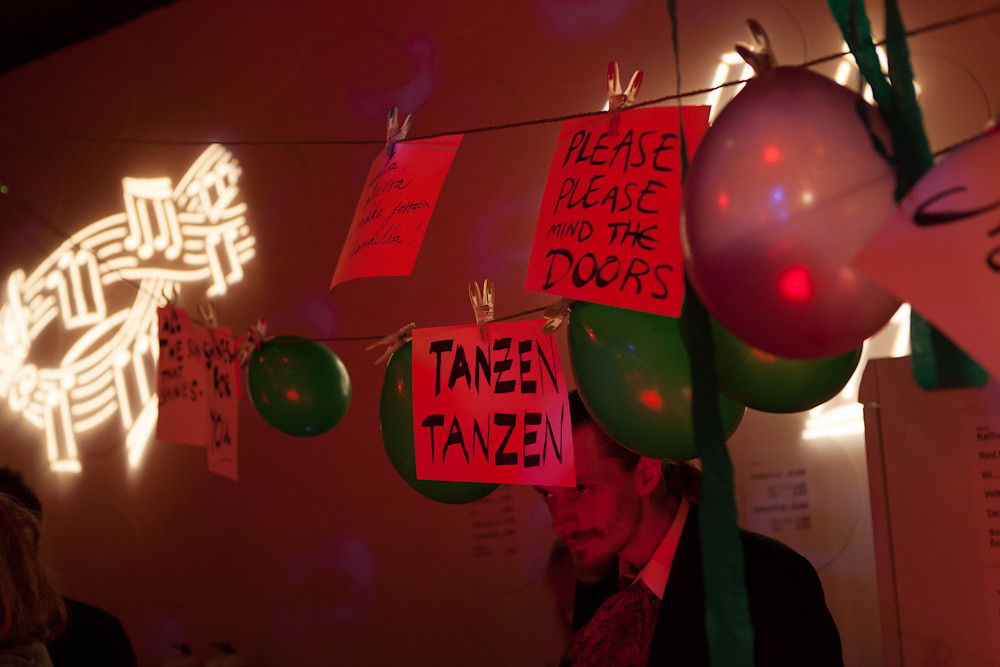In a vividly red-lit room, a man dressed in a formal suit stands beneath clotheslines strung from wall to wall. These lines are adorned with red sheets of paper and colorful balloons—green and pink. Some of the paper sheets display legible messages such as "please please mind the doors" and "Chen Zhen," though others are obscured from view. To the left, a glowing yellow neon sign in the shape of musical notes compliments the scene. The overall ambiance is saturated with red lighting, creating a surreal, almost party-like atmosphere.